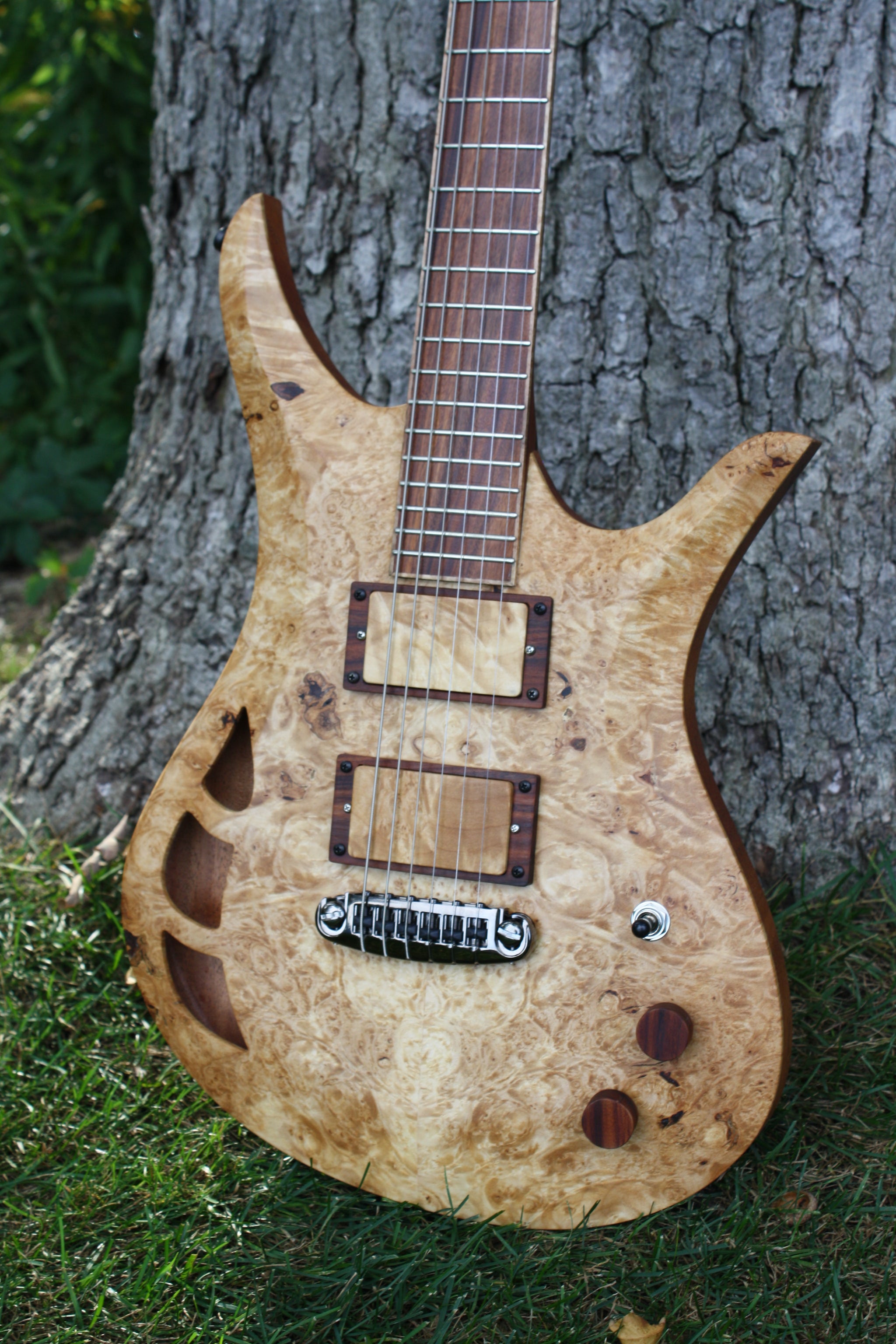This vibrant outdoor color photograph features an electric guitar carefully propped against the lower half of a tree with distinctly gray, rough bark. The guitar, positioned centrally, stands out with its beautifully burled, light wooden finish. The body of the guitar showcases three decorative cut-outs on its left side—two rectangles and one triangle—and is equipped with two dark wooden tuning knobs and an electrical switch on the bottom right. Its strings run down the dark wooden neck, though the headstock is not visible in the frame. Surrounding the tree and at the guitar's base is a neatly manicured, sunlit patch of green grass, accompanied by some additional greenery in the background, giving the scene a serene and well-maintained appearance, likely captured on a pleasant summer day.